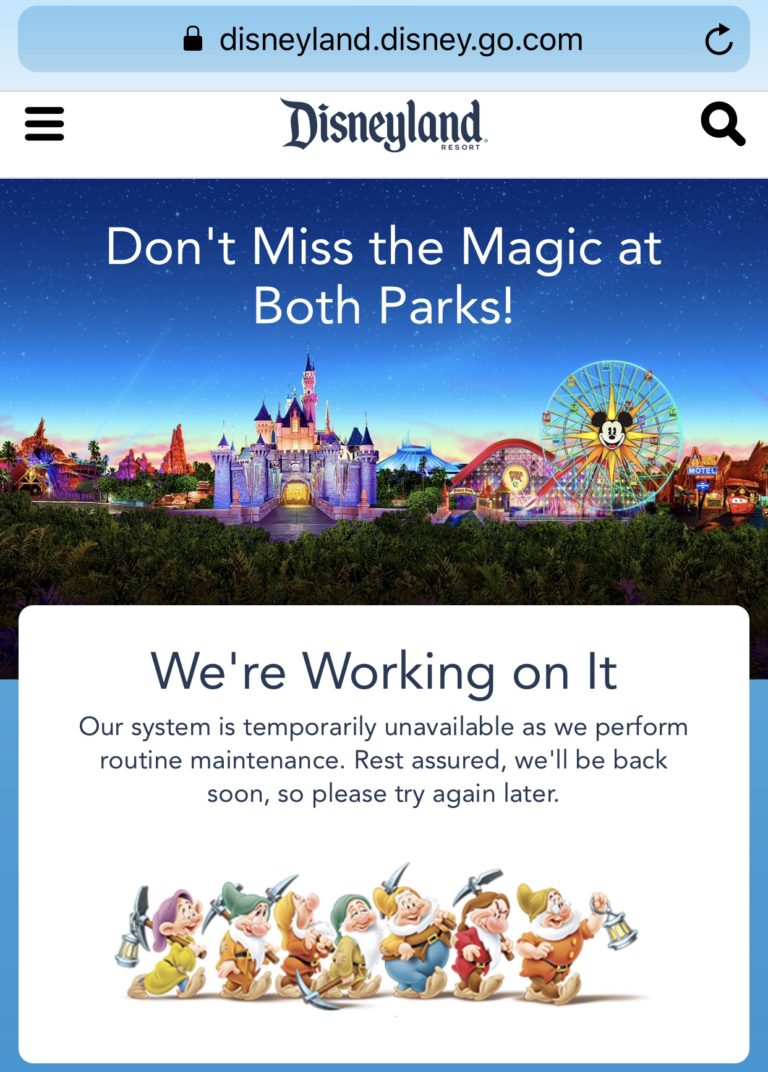The image from the Disneyland Resort website showcases a message indicating that the system is currently down for maintenance. At the very top, the website URL is displayed: Disneyland.Disney.Go.com, accompanied by an option to refresh the page. The Disneyland Resort logo is prominently featured, flanked by a hamburger menu icon on the left and a search magnifying glass on the right.

Beneath the header, a vibrant image captures the enchanting atmosphere of Disneyland, highlighting iconic castles, thrilling roller coasters, and other attractions set against a clear blue sky adorned with twinkling stars. Above this picturesque scene, a cheerful message reads, "Don't miss the magic at both parks."

Just below the image, a notice informs visitors that the system is temporarily unavailable due to routine maintenance. It reassures users that service will resume shortly and encourages them to try again soon. Adding a whimsical touch, the Seven Dwarfs are depicted marching with tools in hand, symbolizing the ongoing efforts to restore the site. Trees border the fantastical landscape of Disneyland, completing the captivating and reassuring message that the magic will soon return.